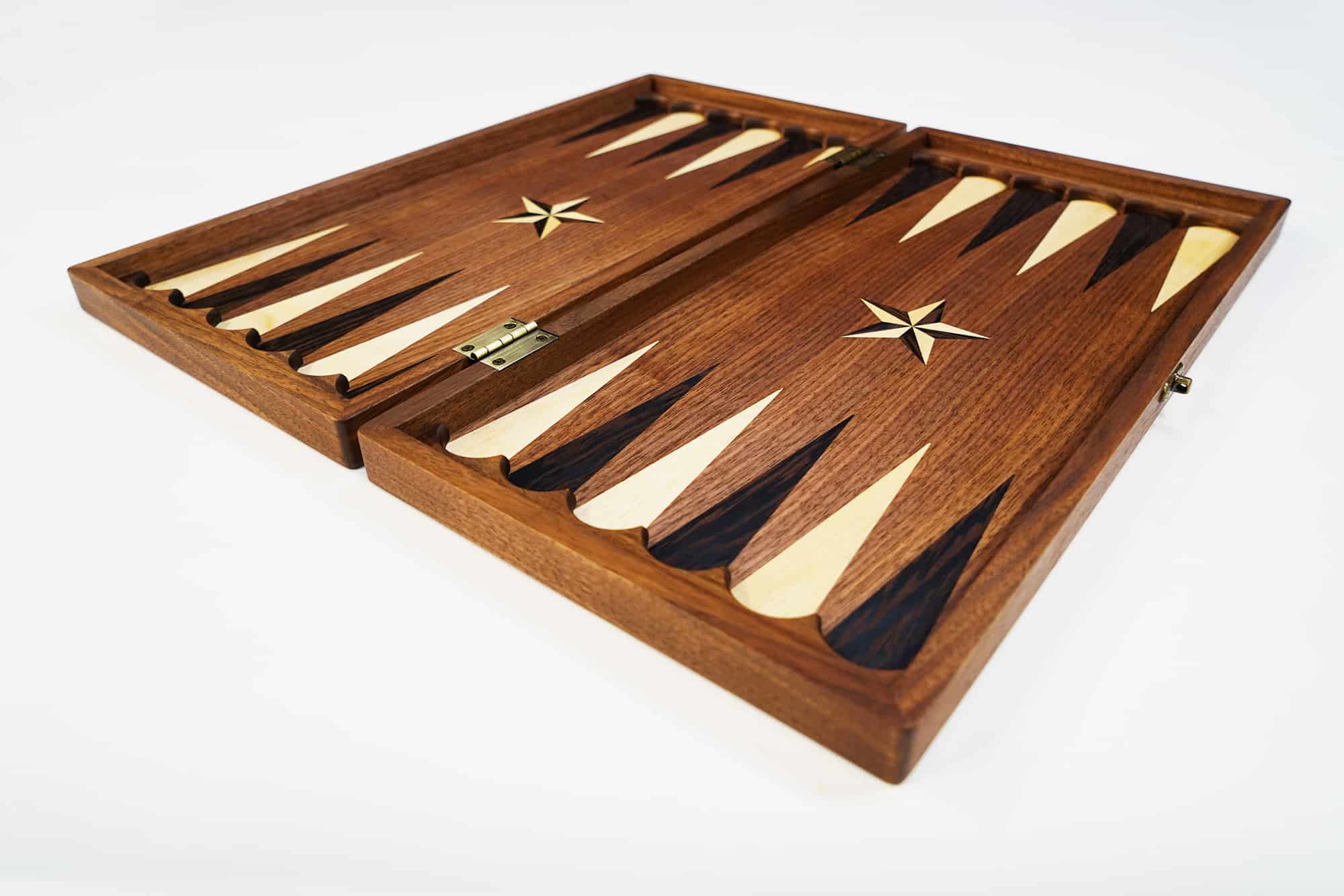This photograph features a dark caramel-colored wooden game board resting on an off-white surface. The board appears to be a hinged, foldable design, held together by a light gold hinge situated at the center. The wood is intricately carved with patterns, including alternating black and off-white triangle shapes across both sides of the board. Each side of the board also displays a central star motif in dark brown and off-white. To one side of the board, there's a round, metallic, gold-colored object, possibly related to the game. The overall composition highlights the craftsmanship of the wooden board and the detailed carvings that adorn it.